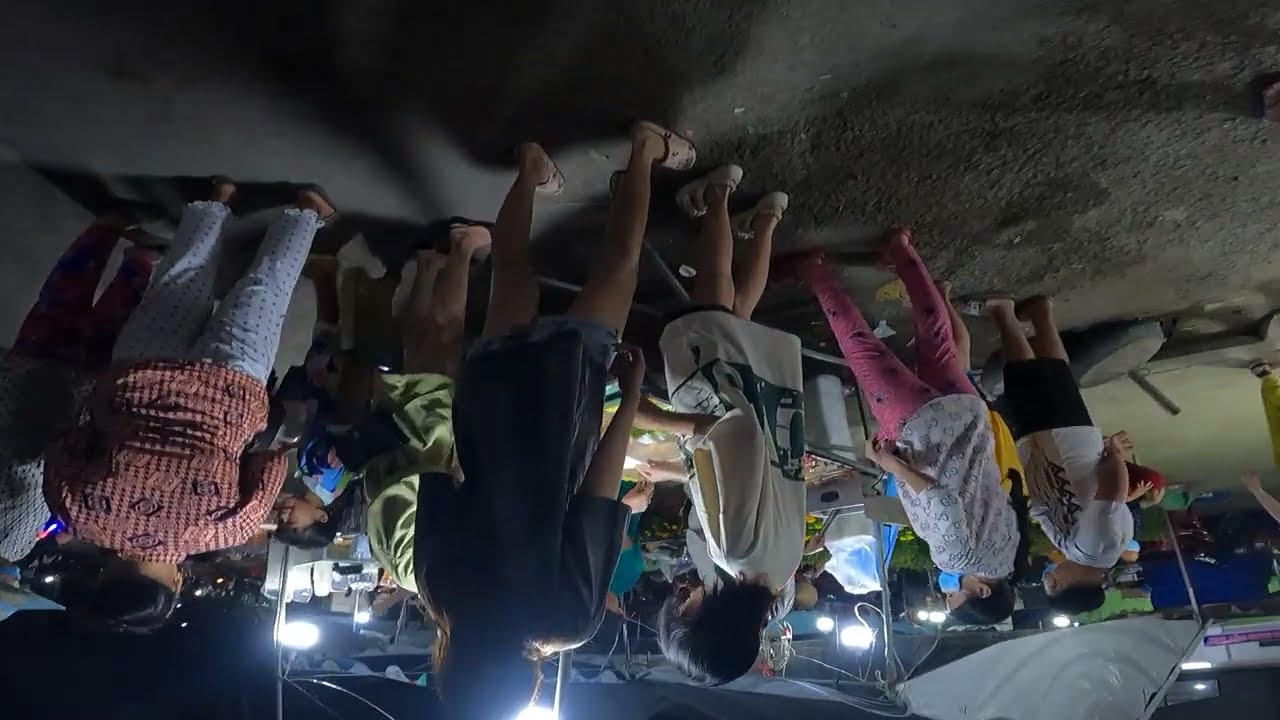The photograph, presented upside down, captures a diverse group of people standing outdoors on a dark, concrete surface, possibly resembling a dirt pathway or asphalt. Despite the flipped orientation, visual details suggest this scene takes place during the night under bright lights, illuminating the background, which features white tents adorned with pastel-colored triangular flags, hinting at an outdoor festival setting. The individuals, mostly of Asian descent, are dressed in various attire indicating temperate weather: some in long-sleeved shirts and pants, others in shorts and t-shirts, with many sporting Crocs and a few wearing face masks. A particular detail includes some people looking away from the camera, engaging with the scene or activity under the tents, potentially involving food or vendor interactions. The overall atmosphere is slightly disorienting due to the upside-down presentation but suggests a lively, communal nighttime event.